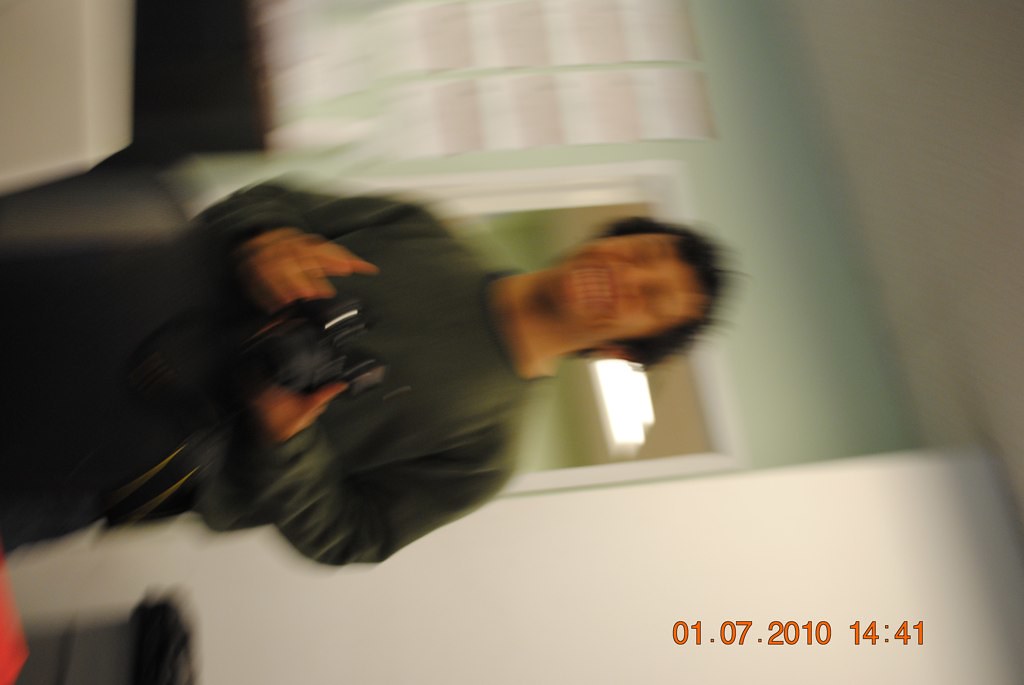This photograph, taken on January 7, 2010, at 2:41 PM, is a heavily blurred, sideways image of an individual with dark, curly hair. The person appears to be holding a camera and is dressed in a dark green sweatshirt and dark pants. The wall behind them is painted in shades of white and mint green. Due to the blurriness, the person's facial features are distorted, giving the illusion of multiple rows of teeth. In the background, a dark garbage bag is visible in a waste bin, positioned next to a series of windows and a single door.